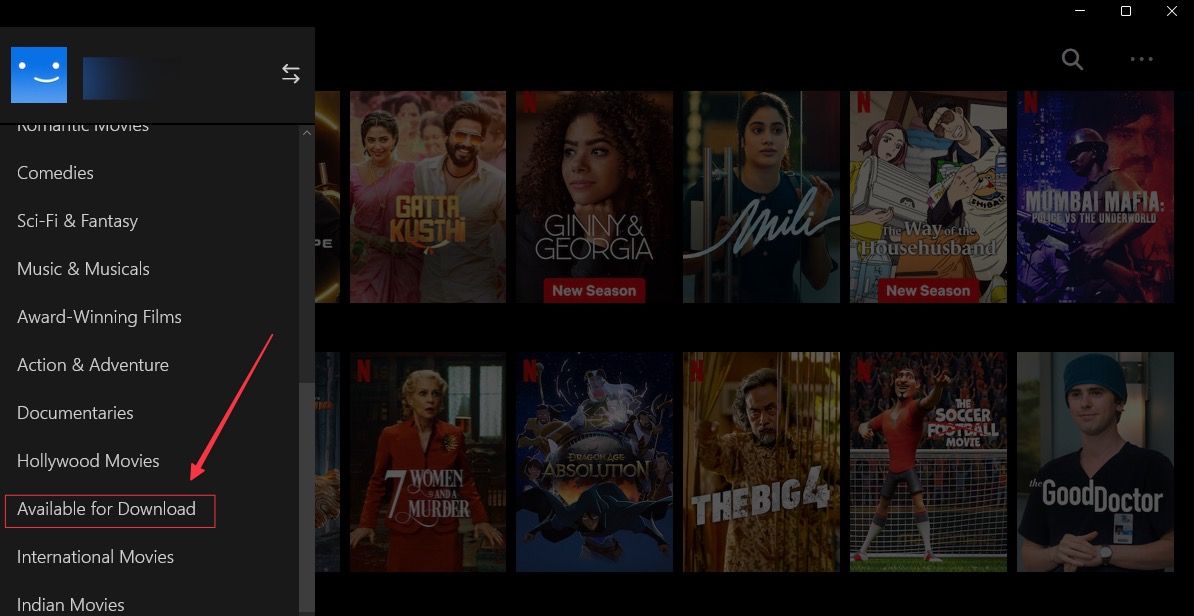The image captures a Netflix library interface, showcasing a diverse selection of movie genres. Located at the top left corner, the profile icon menu is open, allowing users to switch between different Netflix accounts. The selection menu extends horizontally from left to right beneath the profile icon, displaying various categories. The categories listed include "Romantic Movies," "Comedies," "Sci-Fi and Fantasy," "Music and Musicals," "Award-Winning Films," "Action & Adventure," "Documentaries," "Hollywood Movies," and more.

Highlighted prominently in a red box is the "Available for Download" category, with a red arrow pointing to it, indicating user focus. Further categories visible include "International Movies" and "Indian Movies." On the right side of the image, a series of movie thumbnails is displayed, providing visual previews of the available titles within the selected category. The layout is user-friendly, designed to offer a seamless browsing experience for Netflix users.